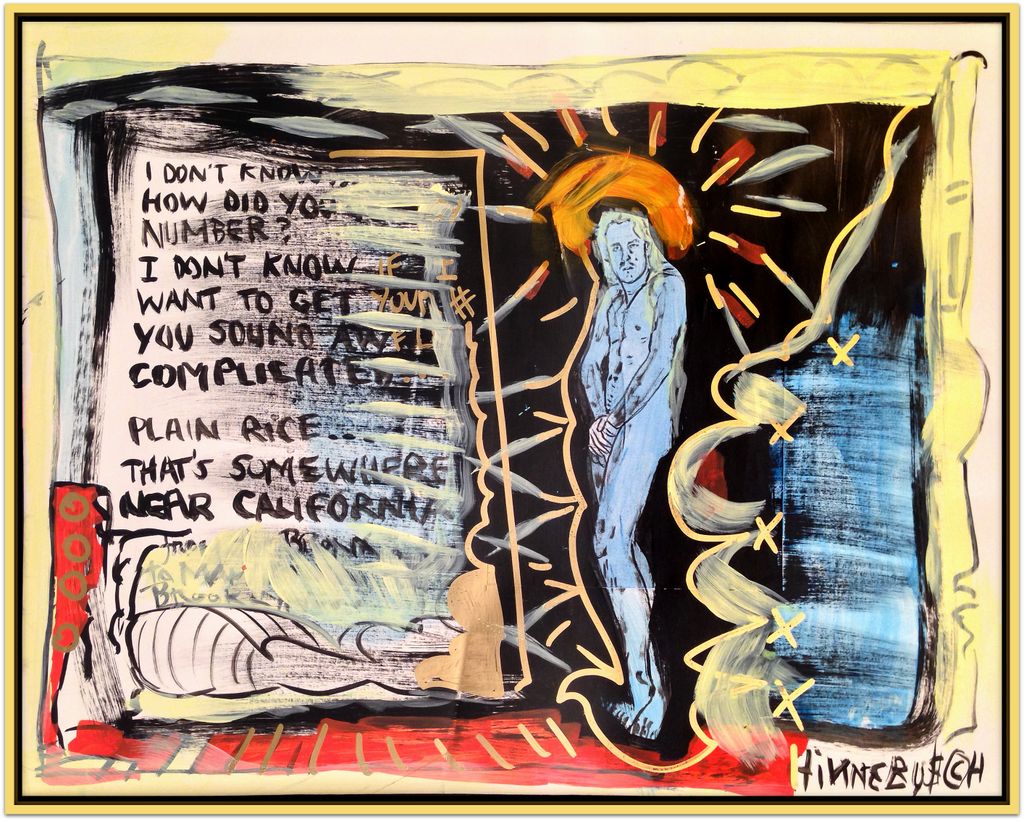The painting features a striking central figure, a naked man depicted in a bluish hue with long hair and a faint mustache. Adorned with a necklace bearing a cross and surrounded by a radiant, large halo emitting white beams, the man's posture is humble, with hands clasped near his crotch. To his left, text is scribbled haphazardly on what appears to be a leaf-like pamphlet, stating phrases like "I don't know how do you number," "I don't know if I want to get your number," "you sound awful," "complicated," and "plain rice. That's somewhere near California,” though much of it is obscured by scribbles and paint. Adjacent to the man's right is a mysterious blue box, accentuated with a yellow line and fluffy movement, adorned with X's, which connects to the man’s halo and an encompassing border. The bottom of the painting features the name "HINNEBUSCH" and a vibrant red flower with brown strands and golden strips, adorned with parallel lines. The entire scene emits an ethereal and unusual aura, interweaving religious and cryptic modern elements into a single, captivating composition.